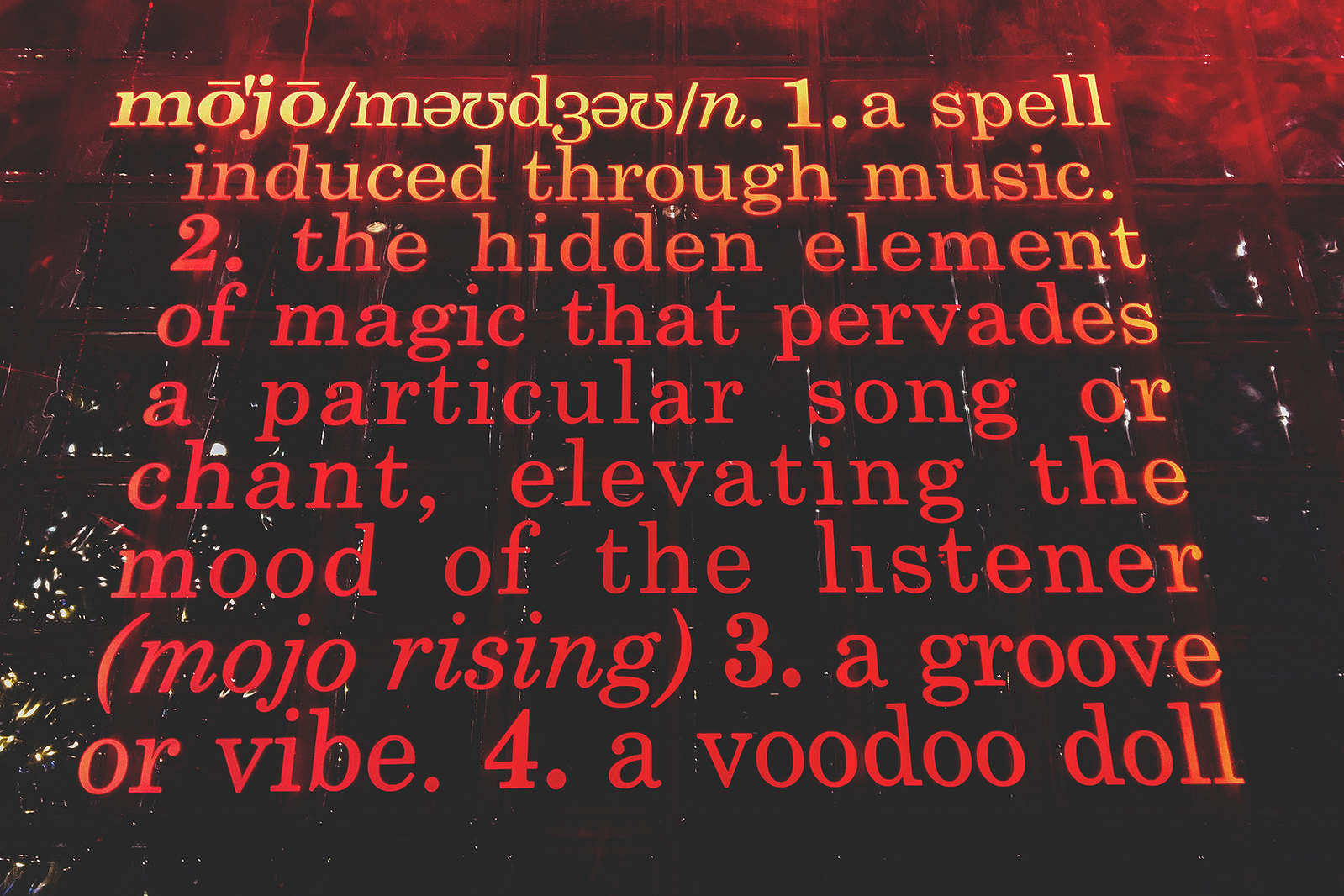The image features a black background with a reddish tint, resembling the appearance of a glass or tiled wall. Dominating the frame is the word "Moho" in a striking yellow and red gradient font, presented as if in a dictionary entry. Detailed phonetic symbols and the abbreviation "N." for noun follow the term. Below, four definitions are listed in a gradient of yellow to red text: 1) a spell induced through music, 2) the hidden element of magic in a song or chant that elevates the listener's mood, accompanied by "Moho rising" in parentheses, 3) a groove or vibe, and 4) a voodoo doll. The image aims to convey the mystical and multifaceted nature of the term "Moho."